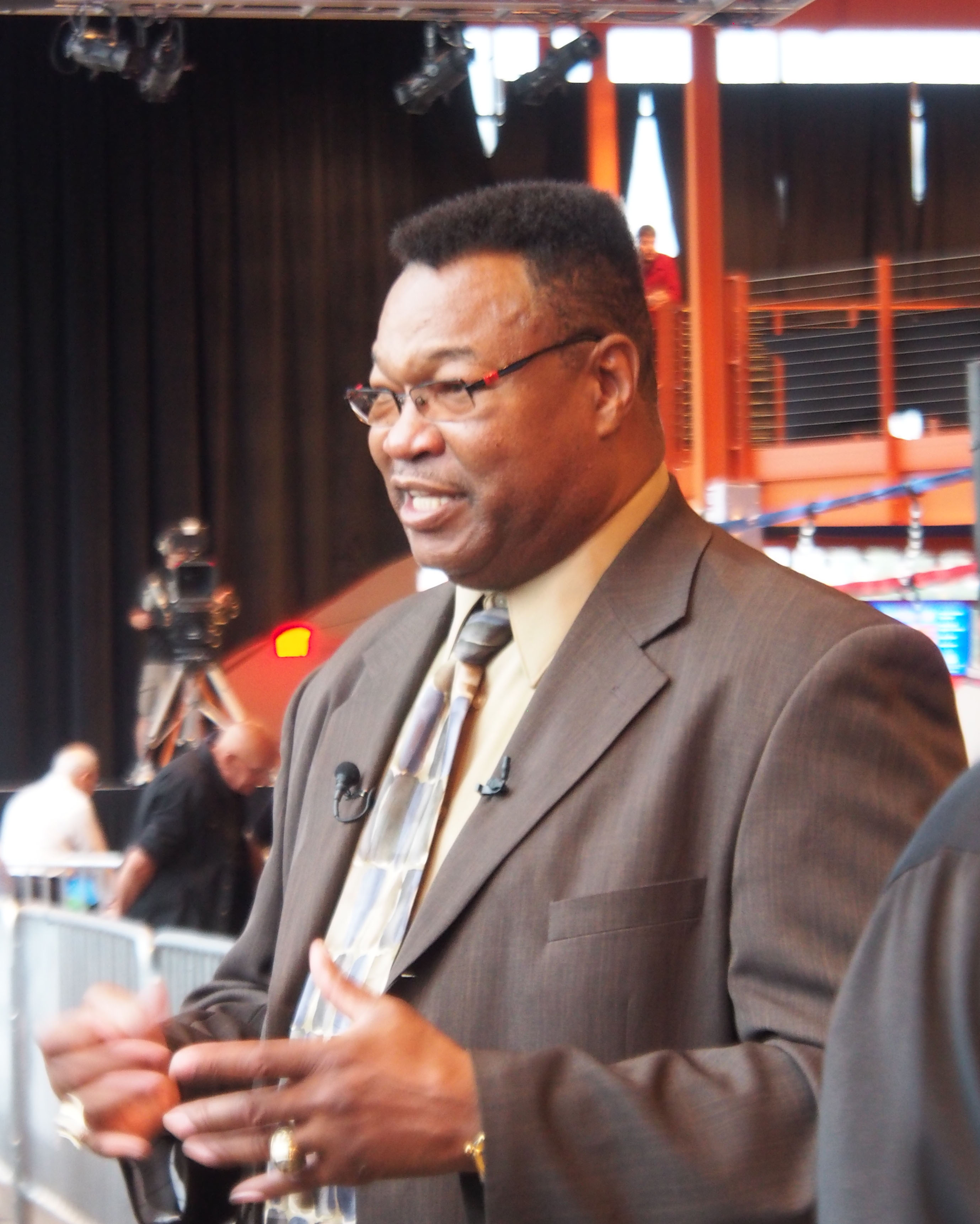In the image, a richly draped giant curtain dominates the background, extending across most of the wall. Several ramps and staircases are visible, leading up to multiple floors. At the top, multiple camera crews with their equipment and lights can be seen. At the center of the image, an African American man stands facing slightly to the left, seemingly engaged in conversation with someone just out of frame. The scene is devoid of any text. The colors present include black, white, gray, orange, silver, red, blue, and gold. The overall setting appears to be a semi-indoor event space, likely a location where some form of filming or production is taking place.